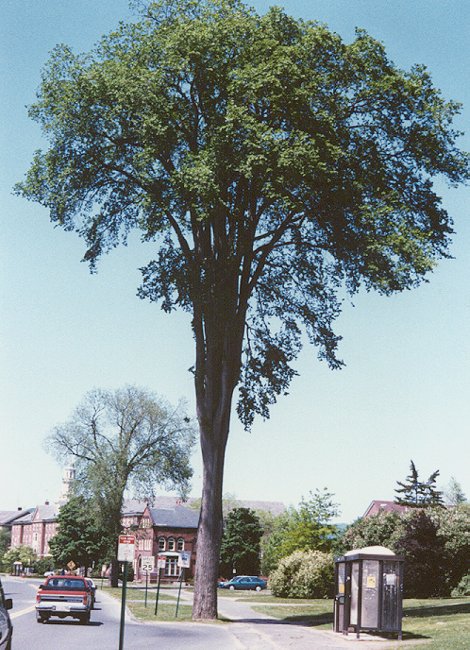This vertically oriented photograph captures an imposing, large tree situated in a residential town setting. The strong, grayish trunk of the tree extends upward from the bottom center of the image, with its branches spreading out vertically and arching into a lush canopy of green leaves against a gradient sky that transitions from blue at the top to white near the base. To the right of the tree, a glass and metal-framed bus stop, complete with a rectangular trash can, sits adjacent to a gray sidewalk bordered by grass. Flanking the two-lane street to the left of the tree are three street signs, including a clearly visible 25-mile-per-hour speed limit sign. Several cars are parked and driving along the road. In the background, past some smaller bushes and trees, stands a large brick building with a structure resembling either a hotel, church, or academic institution, adding to the serene yet bustling ambiance of the scene. The predominant colors in the photograph include variations of green, gray, light blue, black, brown, and white, with all elements positioned upright within the vertical frame.